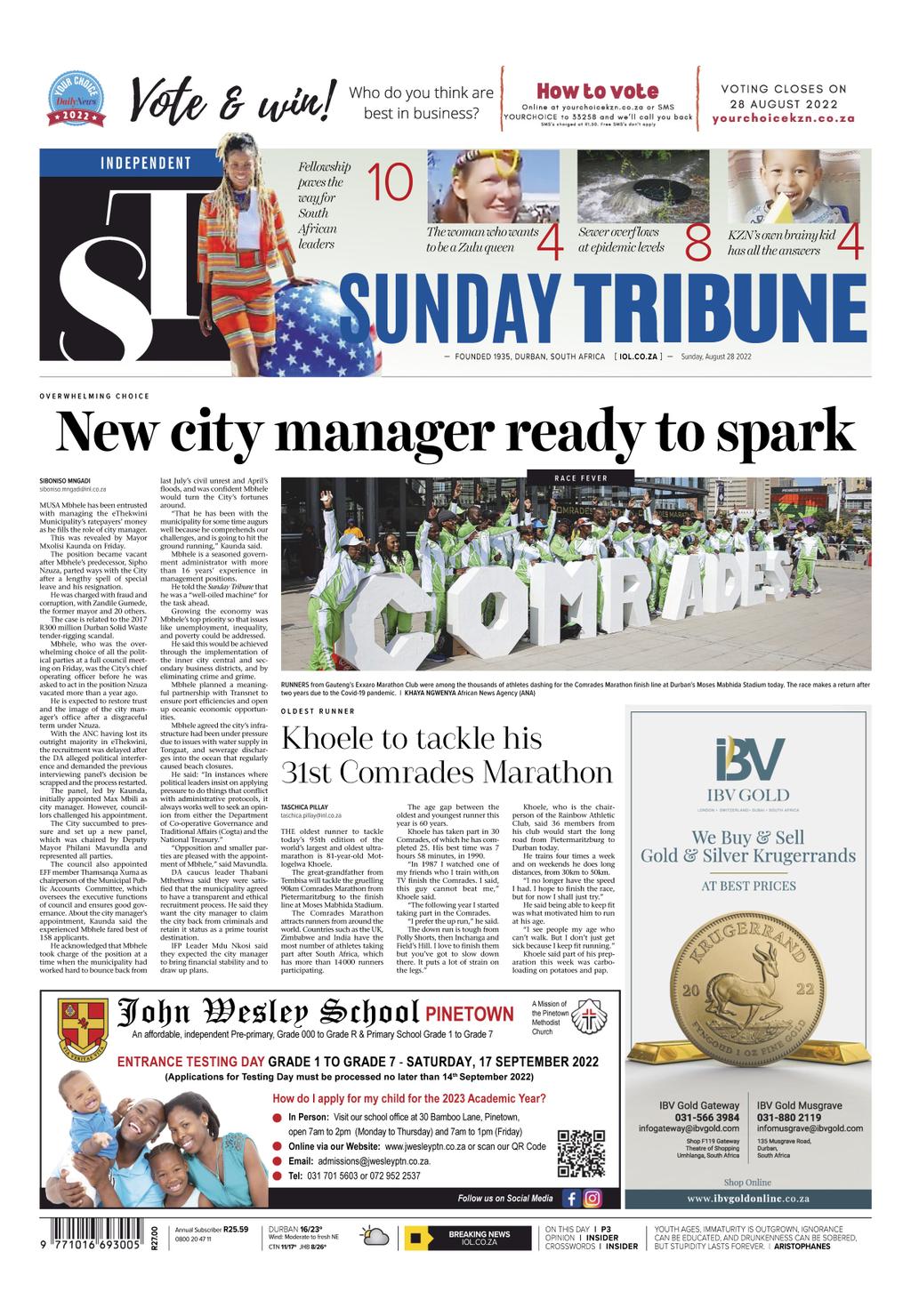This is a detailed descriptive caption for the provided screenshot:

---

Screenshot of the front page of a newspaper. In the upper left-hand corner is the newspaper's logo. To the right of the logo, in black curved text, the headline reads "Vote & Win!" with an exclamation mark at the end. Three light gray arrows point across the top of the page, each with accompanying text. Below this section is a distinct rectangular area. On the left side of this rectangle, a black background houses the white, all-caps letters "ST," with the "S" positioned slightly lower than the "T." Above this black section is a blue banner containing the word "Independent" in white. Adjacent to this, on the right, is an image of a woman. Towards her side, a blue ball adorned with white stars is noticeable. Right next to this, in bold blue letters, it says "Sunday Tribune," with the word "Tribune" more prominently bolded. Just below this, the main headline "New City Manager Ready to Spark" is displayed in bold black font. Beneath the headline, columns of the article unfold in black text. To the lower right of the headline is a rectangular photograph labeled "Comrades" in large white letters, with people standing in the background. Further down, a different article headlines "Chloe to Tackle His 31st Comrades Marathon." There are also advertisements placed on the right-hand side and across the bottom of the page.